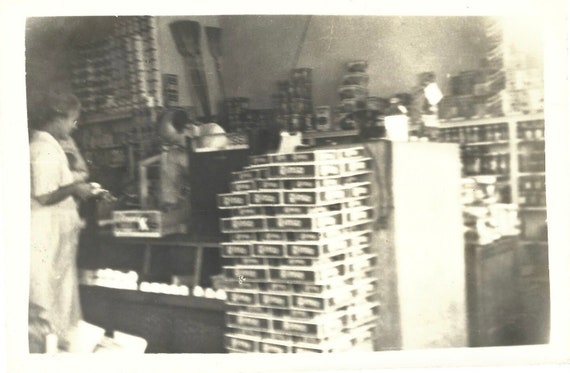This is a black and white photograph, seemingly quite old and somewhat overexposed, contributing to its blurriness and the loss of certain details over time. The image captures the scene inside an old general store or some type of shopping center. In the foreground, we see a man with short hair, bald on top, standing behind a counter. To his left is an old-style cash register. Opposite him, a woman dressed in a long, white dress stands facing him, possibly holding money. The counter is topped with what appears to be a glass case containing various items. Centrally in the picture, a stack of thin, identical boxes with white writing lies on top of one another. The background features shelves stocked with cans, boxes, and tins. To the far left, leaning against the wall, are a pair of brooms. The photograph is light-stricken from the right side, adding to the difficulty in discerning finer details.